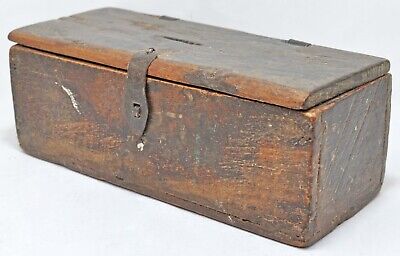In the image, there is a long, rectangular wooden box that appears to be very weathered and aged, suggesting it might be an antique. The wood panels cover all sides of the box, including the lid, which features an iron latch for closure. The box also has an open slit at the top, reminiscent of a slot for coins, making it potentially useful as a piggy bank. The wooden surface is darkened and marked with scratches, gouges, and dark stains, alongside remnants of white paint, indicating extensive use over the years. The box’s lid is hinged at the back to hold it open when required. It sits in front of a plain, light grey background, highlighting its rugged and storied appearance. There is no text in the image.